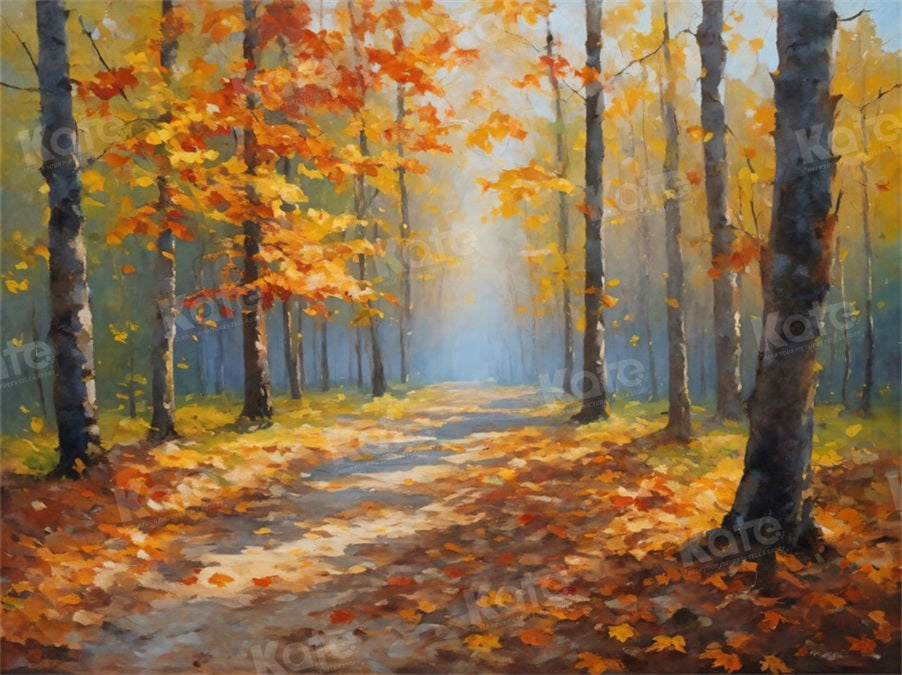This painting depicts a serene autumnal forest scene with a prominent gray pathway running through the center, leading into a lush, colorful landscape. The trees, varying in vibrant shades of yellow, orange, and red, flank both sides of the path, their dark brownish-gray trunks adorned with black spots reaching up toward a light bluish-gray sky. Scattered leaves blanket the ground, enhancing the seasonal atmosphere. The sky exhibits a subtle gradient, transitioning from a light blue to hints of sunshine filtering through the foliage. In the background, as the details fade, the scenery blends into a vague blue abyss, giving a sense of depth and distance. A diagonal watermark, the word "KOTE" repeated numerous times, runs across the image from the bottom left to the top right, subtly integrating with the overall composition.